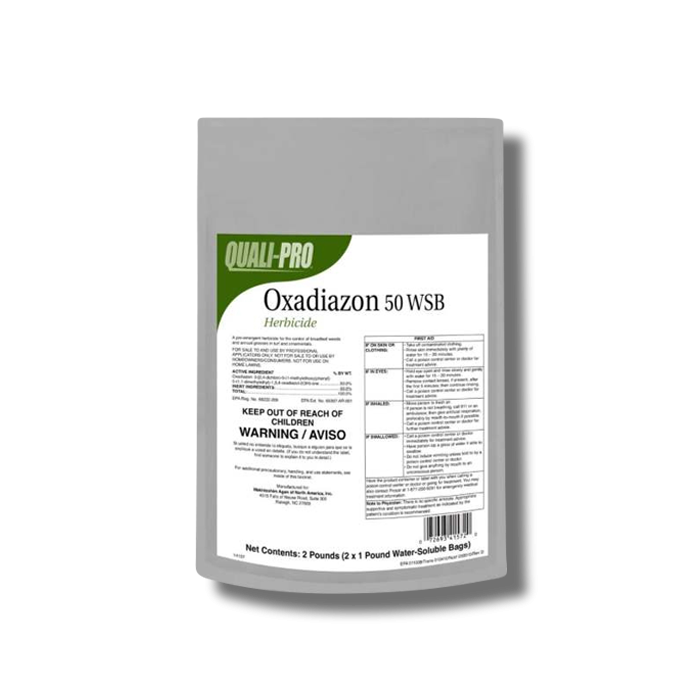The image depicts a label for a herbicide called "Quali-Pro Oxidiazone 50 WSB". The label has a predominantly white background with black text. In the upper left corner, the brand name "Quali-Pro" is displayed against a green background with a curved edge. Below, in bold black text, it reads "Oxidiazone 50 WSB Herbicide". There is smaller, less readable text printed in black that includes a warning, "Keep out of reach of children," and other legal or usage information. On the right side, a simple printed chart is visible, though the text within it is blurry. At the bottom of the label, it clearly states "Net Contents: 2 Pounds (2 x 1 Pound Water Soluble Bags)." Additionally, there is a barcode located in the bottom right corner. The label's simplistic design suggests it is part of a pouch or container.